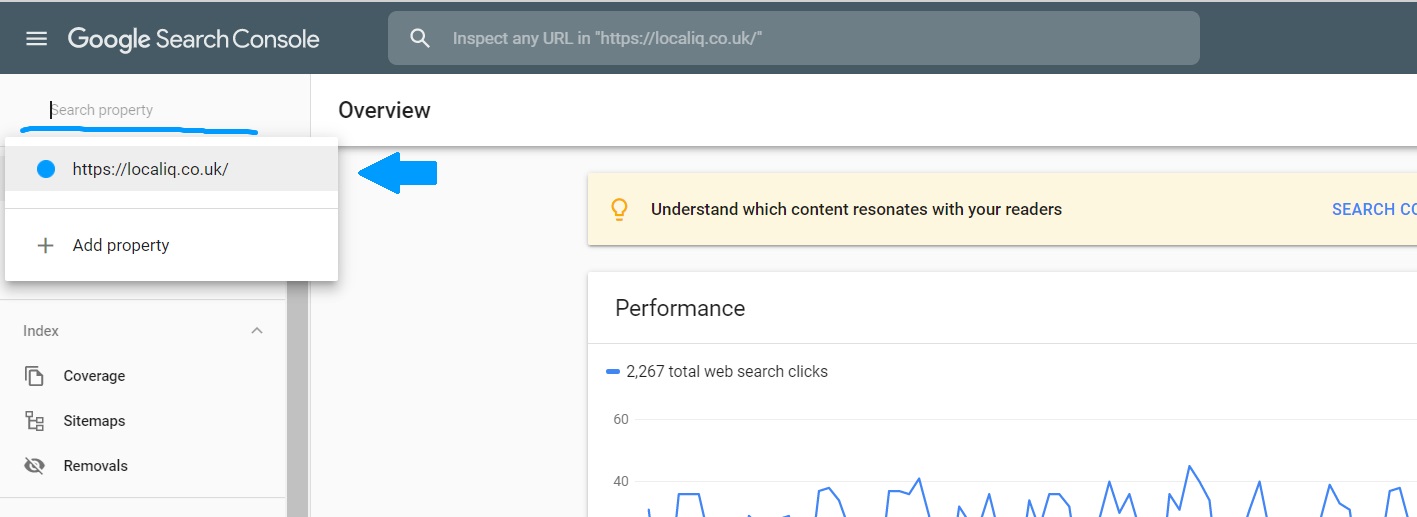This screenshot captures a detailed view of the Google Search Console interface. At the top, the medium gray horizontal bar features three white horizontal lines on the left, followed by the text "Google Search Console." To the right, a search bar with a light gray background includes a white magnifying glass icon and the placeholder text "Inspect Any URL in HTTPS://localIQ.co.uk/."

Underneath, the interface displays a search property box on the upper left with a blinking cursor, indicating it's actively being used. This box is highlighted with a hand-drawn blue underline and shows one result in a pop-up list. The result features a blue circle, the URL "HTTPS://localIQ.co.uk/" against a light gray background, a thin dividing line below, and a plus symbol beside the "Add property" option.

On the left side of the console, the navigation column shows an expanded "Index" menu, identifiable by an upward-pointing arrow. This section includes three options: "Coverage" (represented by an icon resembling a sheet of paper with a corner folded), "Sitemaps" (symbolized by a flowchart icon), and "Removals" (depicted with an eye icon with a line through it).

The main interface is straightforward, displaying the text "Overview" at the top. A thick, blue, hand-drawn arrow points left towards the pop-up box. Nearby is an informational box shaded in pale beige or yellow, containing a light bulb icon and the message "Understand which content resonates with your readers." Partially visible is a blue text segment reading "search CO."

Below this, a performance graph is partially displayed, featuring a blue line and the text "2,267 total web clicks" to its right. The graph shows the peaks of a jagged line chart, but the lower part of the chart is cut off from view.